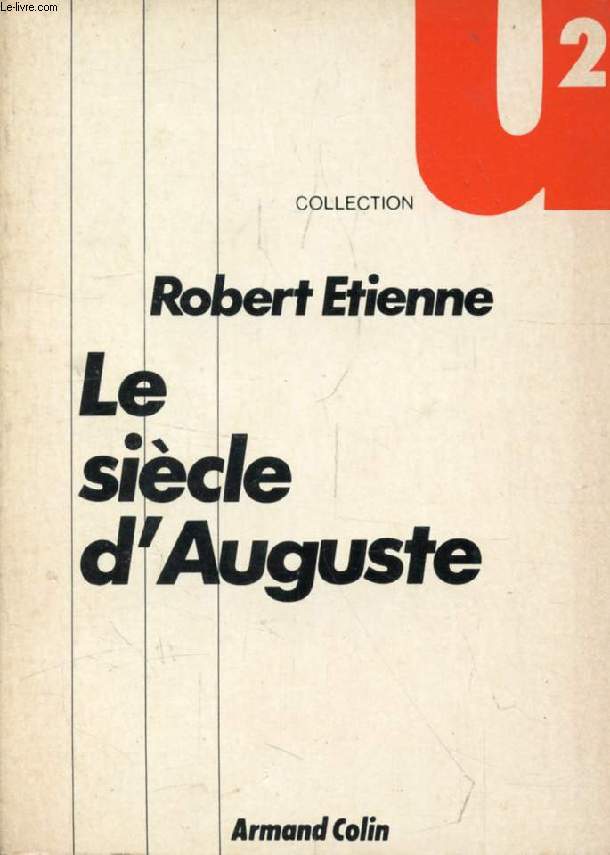This image appears to be the front cover of a book or a music album with a retro and somewhat worn aesthetic. The background is primarily white and appears scratched or aged, giving it a vintage feel. Prominently featured in bold black lettering is the name "Robert Etienne," accompanied by the title "Le Siècle d'Auguste" below it. The text is predominantly in a different language. Additional words include "Collection" and "Armand Colin" centered at the bottom. In the top left corner, there is a web address, LE-LIVRE.com, while the top right showcases a distinctive U2 logo with an orange 'U' and a transparent '2' overlaying it. The primary colors used in the image are tan, black, gray, and red, contributing to its retro style. Vertical lines add to the design along the side of the cover.